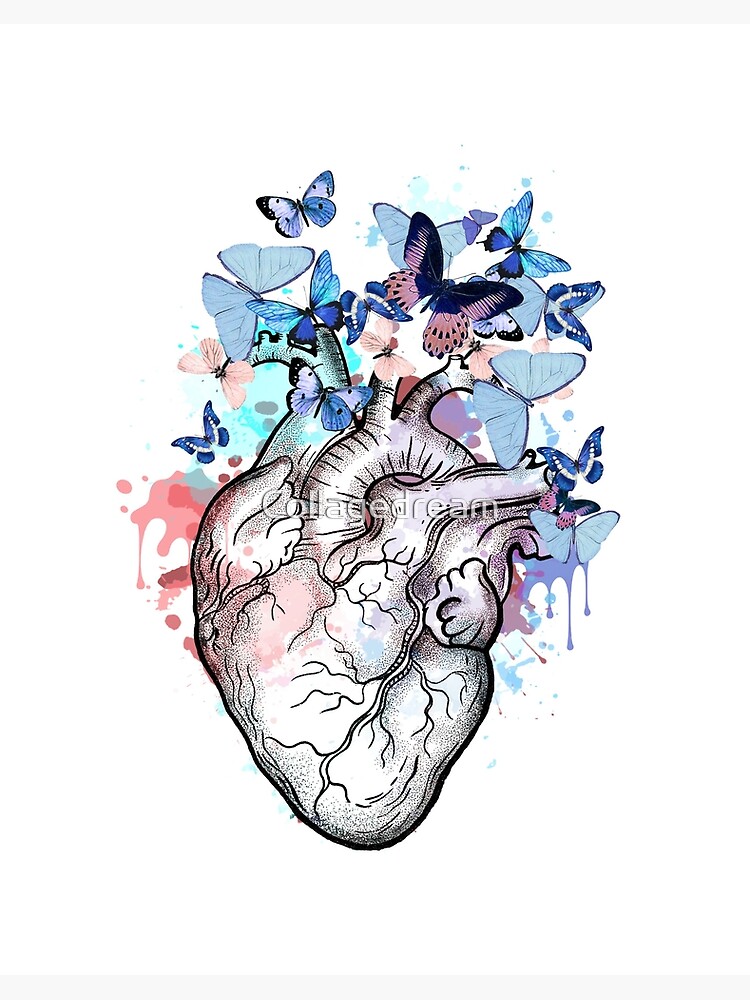The image is a detailed artistic rendition of a human heart, colored primarily in shades of white and some faint pinkish tones, with various veins and arteries prominently depicted, including the aortic arch, the inferior vena cava, and the superior vena cava. The background is white, with a grainy texture providing shading to the heart. Above the heart, there is a vibrant collection of butterflies in various shades of blue, ranging from light blue to teal and dark blue. Additionally, there are a few pink butterflies and one distinctive butterfly with black and pinkish wings adorned with small black spots. The overall scene is accentuated by colorful splatters of red and blue, giving it a unique, dream-like quality. Written faintly across the image in italic script are the words "collage dream," adding an enigmatic and whimsical touch to the illustration.